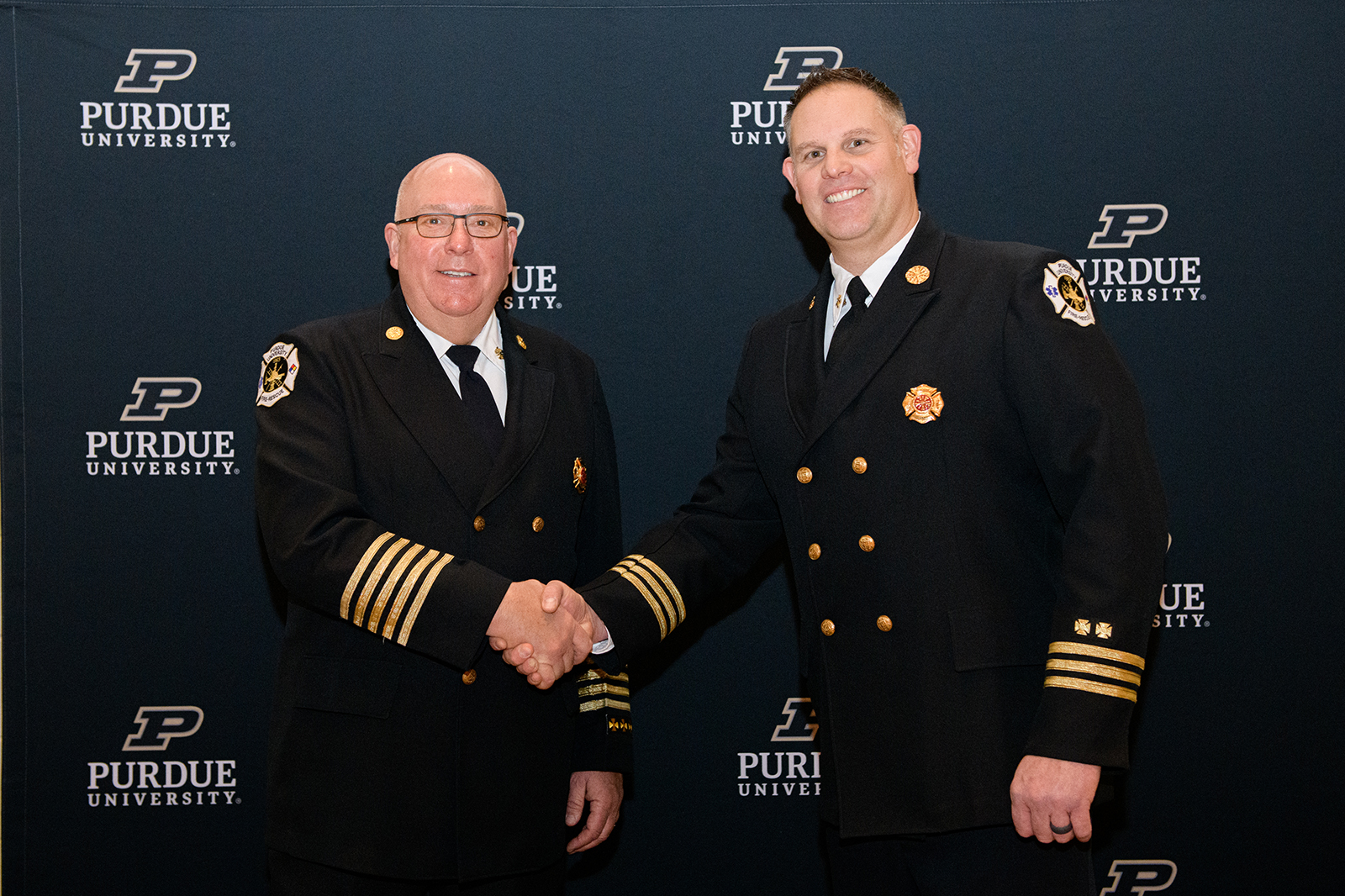This photograph features two middle-aged Navy men shaking right hands while smiling warmly at the camera, teeth showing. The man on the left is noticeably older, in his 50s or 60s, with balding hair and glasses, while the man on the right is likely in his 40s, with short brown hair possibly flecked with gray, and wears a wedding ring. Both men are dressed in identical black double-breasted blazers adorned with gold buttons, gold stripes at the sleeve cuffs (three on the older man and five on the younger), and gold shield-like brooches on their left chests. Their uniforms also feature gold symbols patched on the sleeves. The backdrop is a navy blue billboard with "Purdue University" and the letter "P" repeatedly printed in white, adding an academic tone to the image. Despite the lack of context about the occasion, their happy demeanor and formal attire suggest a celebratory or official moment at Purdue University.